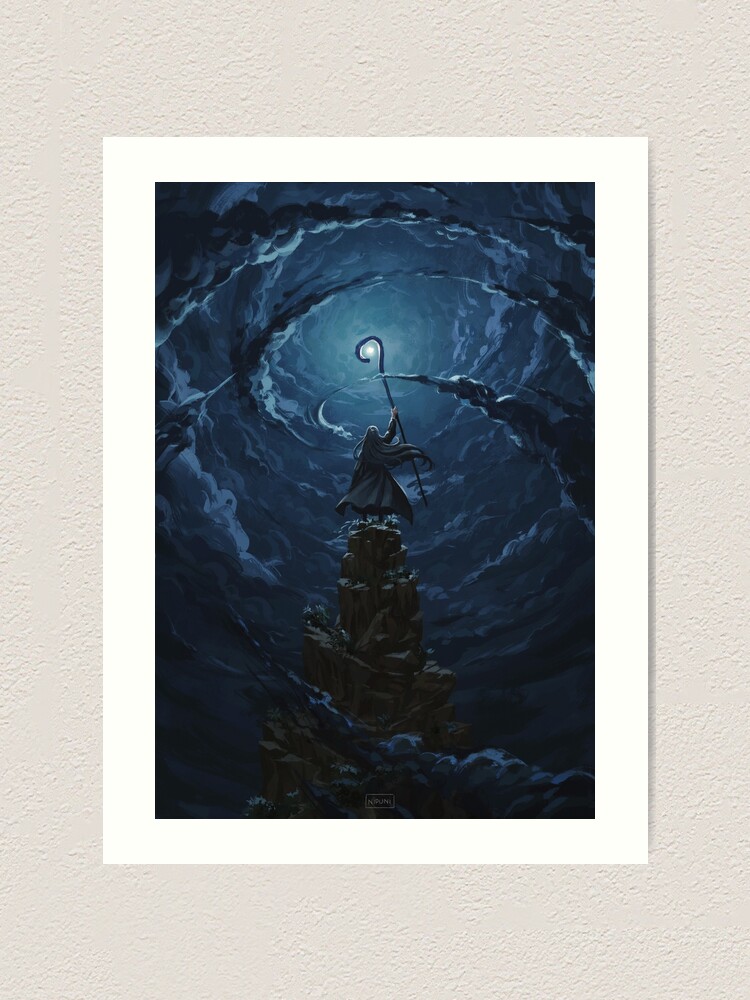The image appears to be a detailed, artistic, watercolor-style painting or AI illustration, prominently framed by a two-inch white border and matted on a khaki background about three to four inches wide. The central image is dominated by a deep, charcoal blue, almost tempestuous sky, with swirling clouds that envelop a rugged, craggy mountain or coral-like structure. At the peak of this rocky formation stands a mysterious figure, seemingly a sorcerer or wizard, with long gray hair flowing from beneath a dark, hooded cloak. The figure's back is turned to the viewer and he holds an imposing, staff-like wand aloft. The top of the staff curves like a hook, perfectly framing the moon in the distance, which faintly lights up the stormy surroundings. The overall mood of the piece is dark and ominous, evoking a sense of foreboding power and malevolent magic as the clouds and sky churn tumultuously. The artist credited appears to be Nippuni, although the watermark is indistinct.